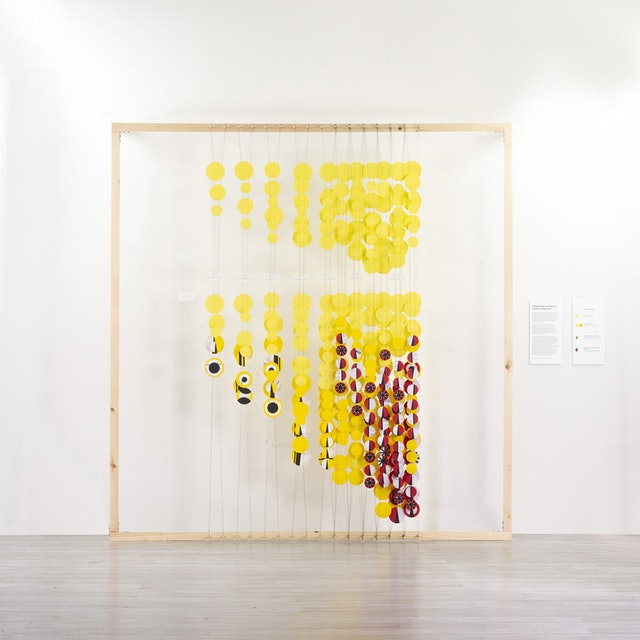The image captures a modern art installation set within an art gallery. The scene is dominated by a thin, light-colored wooden frame that stands against a blank white wall. This frame spans almost the entire height from the floor, which takes up the bottom 20% of the image and is depicted in gray, up to the wall above. Suspended from the top of the frame are multiple vertical strings or wires, each adorned with numerous yellow circles. The arrangement of these circles varies, with fewer circles at the top section and many more densely packed towards the bottom, especially on the right-hand side. Notably, some of the lower circles feature additional colors, including black, red, and white, reminiscent of Pokéballs from the Pokémon series. 

To the right of the wooden frame, two pieces of paper with black text are affixed to the wall, presumably providing information about the artwork. The overall feel of the piece is that of a modern art exhibit, merging simplicity and complexity through its detailed color placement and minimalist presentation. The installation invites viewers to interpret its abstract arrangement and color choices, adding layers of meaning to the lively yet orderly display.